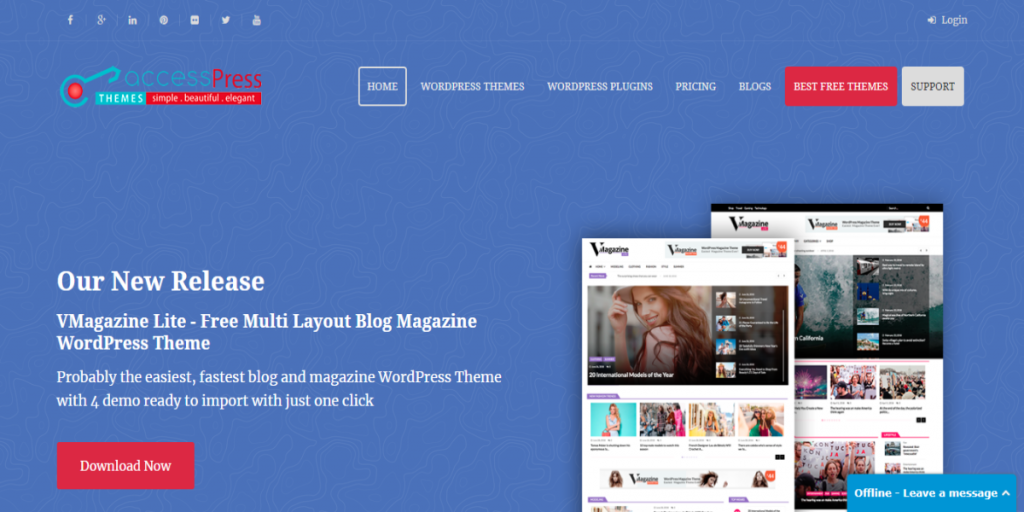The website features a predominantly blue background on the left upper side. At the top left corner, there's an image of a teal-colored key with a red circle in the middle. Beside this image, the words "Access Press" are displayed, with "Access" in light turquoise blue lowercase letters and "Press" in uppercase red letters. Below this, there is a turquoise rectangle with the word "THEMES" inside, written in all capital letters and white text. Adjacent to this is a red rectangle with the same text.

Below are several navigational tabs, with "Home" being highlighted in a square. Other tabs include "WordPress Themes," "WordPress Plugins," "Pricing," and "Blogs." Further to the right, there's a red rectangle with white text saying "Best Free Themes," followed by a white rectangle with black text stating "Support."

Moving to the middle-left section, in white text, it reads "Our New Release V Magazine Lite - Free Multi Layout Blog Magazine WordPress Theme." A subheading states, "Probably the easiest, fastest blog and magazine WordPress theme with four demo ready to import with just one click." Beneath this text, there is a red rectangle with the words "Download Now" in white.

To the right of this section, there are various images depicting the blog magazine theme, including a picture of a woman with long brown hair wearing a hat. The images illustrate different aspects and features of the theme. At the bottom right corner, within a turquoise blue rectangle, it says "Offline. Leave a message" in the center in white text, accompanied by a white arrow pointing upwards.